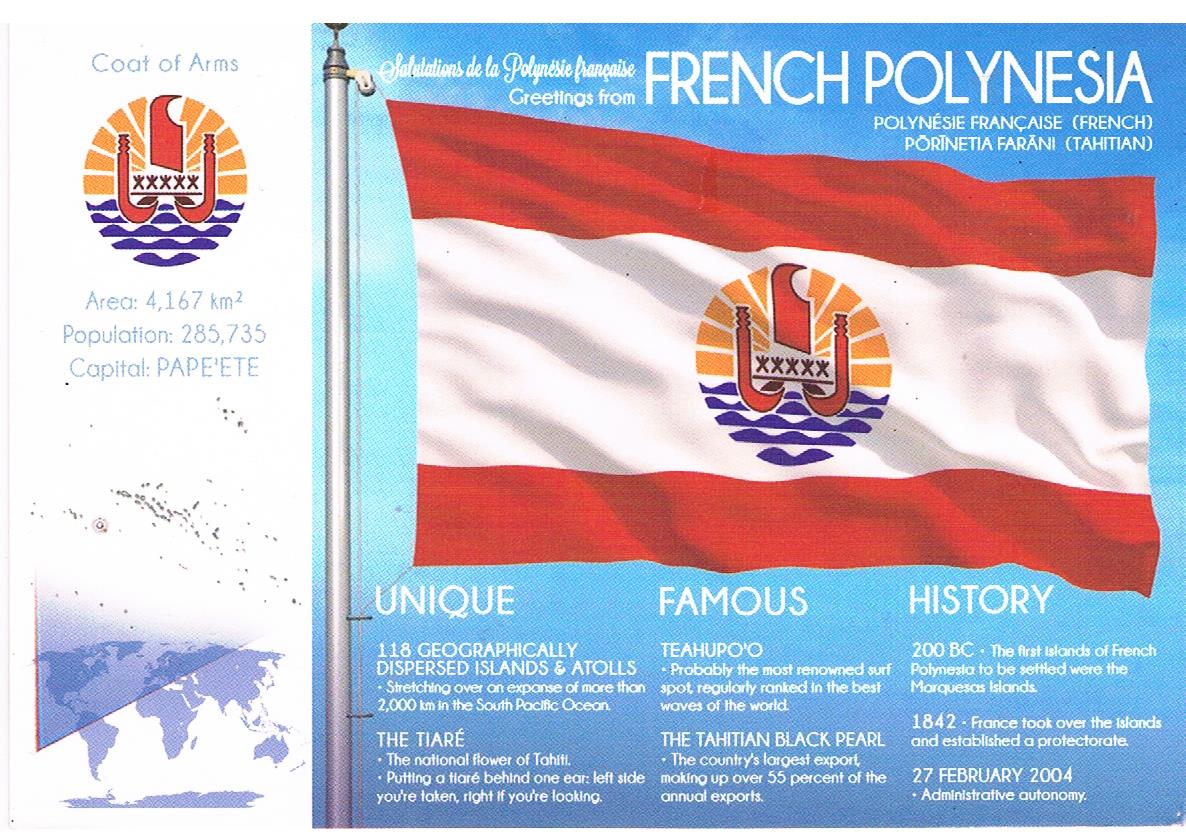The image depicts an advertisement or banner with detailed elements representing French Polynesia. On the left side, occupying about 25% of the image, there's a white vertical banner. This banner includes a coat of arms featuring a circle with a depiction of the sea below and the sun above, colored in orange, red, and light blue. Below the coat of arms, statistics are provided: "Area: 4167 square kilometers, Population: 285,735, Capital: Papeete." A light blue and white world map graphic is also present at the bottom of this section.

The main body of the image showcases a wavy flag of French Polynesia on a blue background. The flag consists of thin red and white stripes at the top and bottom, with a thick white stripe in the middle featuring the aforementioned coat of arms. This flag is accompanied by large, prominent text at the top reading "French Polynesia." Beneath the flag, there is additional text in three columns providing historical facts about the region under the heading "Unique Famous History." The entire presentation appears to be carefully designed to highlight both the visual and factual elements of French Polynesia's identity.